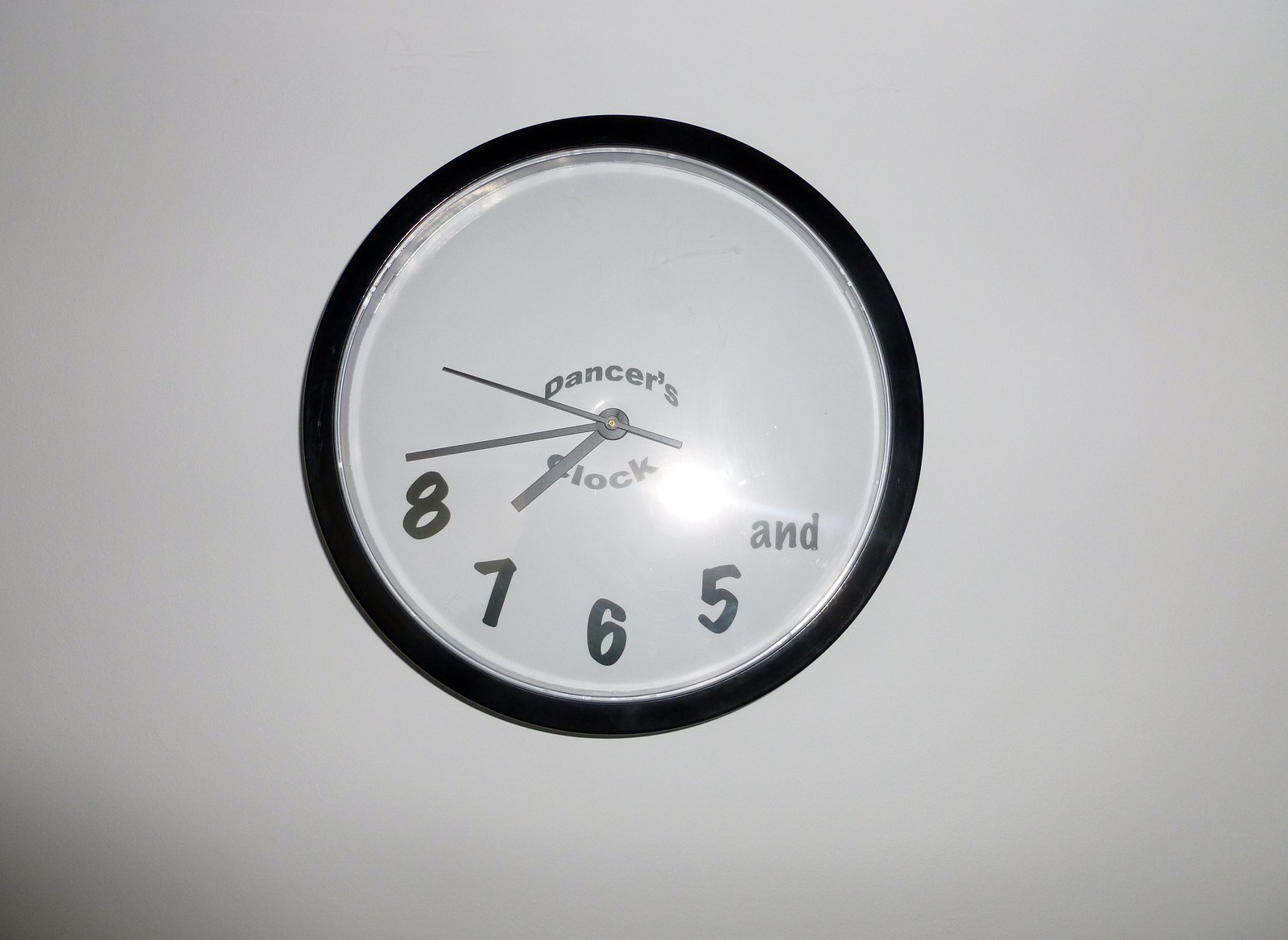This image features a uniquely designed wall clock that prominently hangs on a pristine white wall. The clock is encased in a sleek black rim, framing a stark white face. Instead of displaying the full set of numbers typically found on a standard clock, this one exhibits only the numbers 5, 6, 7, and 8, each positioned in their customary locations on the lower half of the clock face. Above these numbers, the clock is labeled "Dancer's Clock" — a creative nod to the counting rhythm commonly used in dance rehearsals and performances, where instructors count "5, 6, 7, 8" to cue dancers. The clock's minimalist design includes three hands — the hour hand, minute hand, and a second hand — all rendered in a grayish-black hue. The overall aesthetic of the clock is clean and unembellished, emphasizing its playful yet functional tribute to the world of dance.